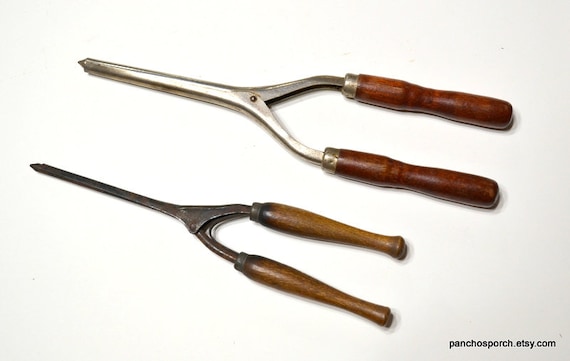The image showcases two vintage tools, reminiscent of old-fashioned pliers or shears, placed against a white background. Both tools have metal fronts that resemble scissor-like points, useful for clamping, pulling, or twisting. The tool at the top features a red wooden handle with silver notches and is noticeably larger and thicker than the bottom tool. The bottom tool, on the other hand, has a beige or dark brown handle with black notches above it. Despite these differences, both tools share a similar design and are closed. The photo also includes a small black font at the bottom of the image, reading "ponchosporch.etsy.com."